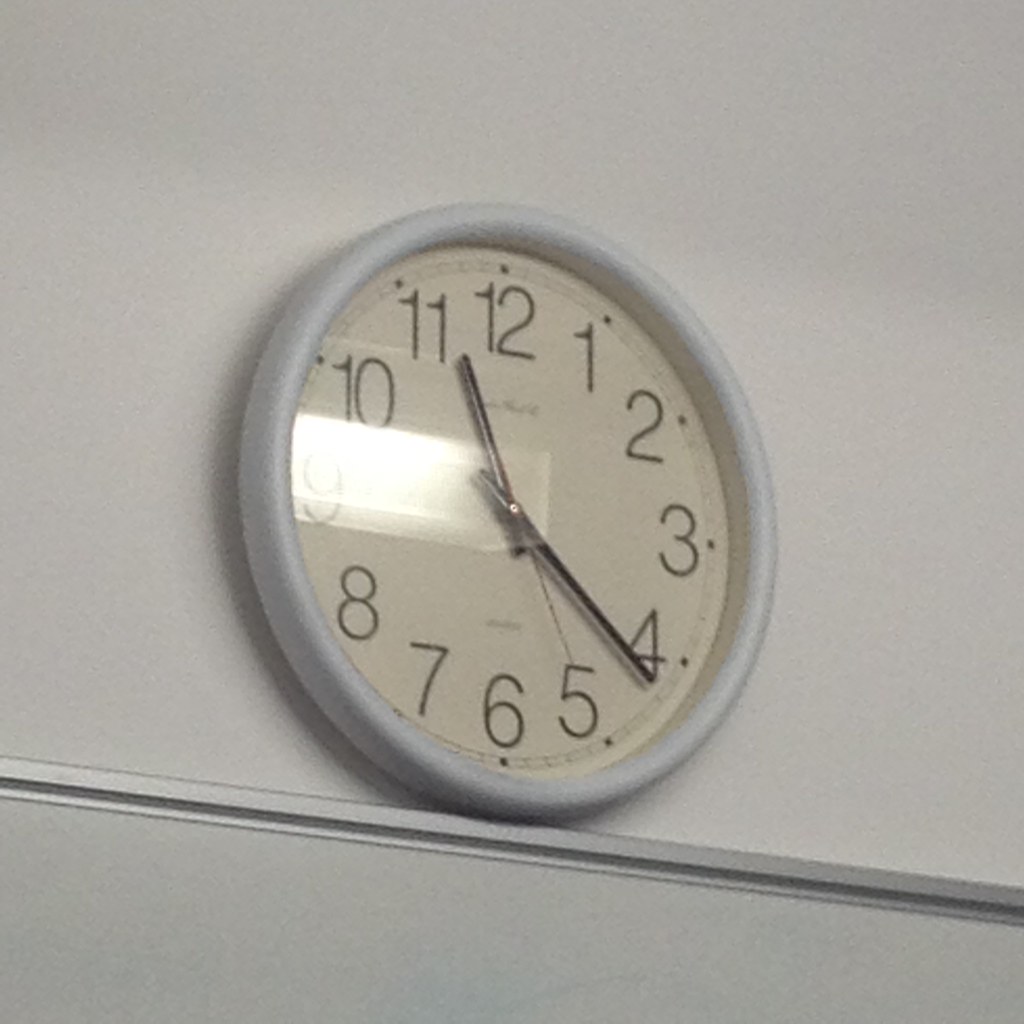This photograph captures a simple wall clock mounted on a bi-colored wall. The wall features a whitish upper section and a greenish lower section, separated by greenish molding. The clock, which sits atop this molding, has a round, white plastic frame with a glass (or possibly plexiglass) cover. The clock face is an off-white, ivory color, adorned with bold, black Arabic numerals from 1 to 12. Each numeral is clear and distinct, and additional writing is visible near the top and bottom within the clock face. The clock is equipped with a simple set of hands—black for the minute and hour, and a silver hand tracking the seconds. The time displayed is precisely 11:22 and 25 seconds. The lighting casts a slight shadow from the upper right, hinting at an overhead fluorescent box light, possibly from a classroom setting. The clock face also reflects this light, adding to the photograph's detailing. All elements combined create a meticulous and well-lit image of a utilitarian clock against a contrasting two-toned wall.